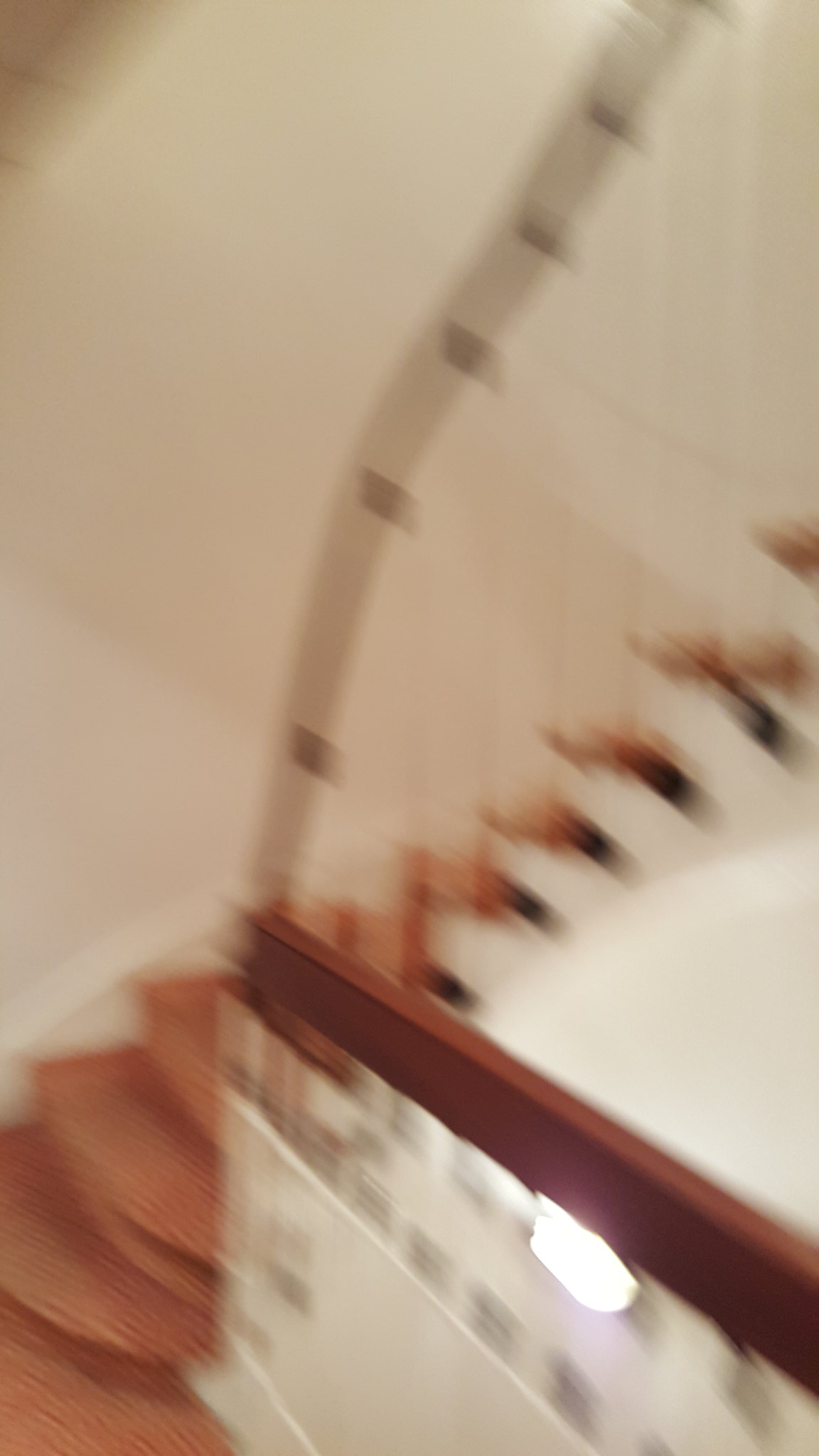The photograph captures a spiral staircase, though the image is rather blurry and out of focus. Dominating the bottom right corner is a banister featuring a burnt orange-brown railing contrasted by a white section underneath. The background on both the left and right sides reveals white walls. The staircase itself is adorned with an orange carpet, which appears spotty, possibly due to the blurriness, suggesting a mix of orange and white spots. The steps begin at the base and curl upward, with the sides appearing darker than the center. A corresponding railing accompanies the staircase, adding to the structure's intricate design.